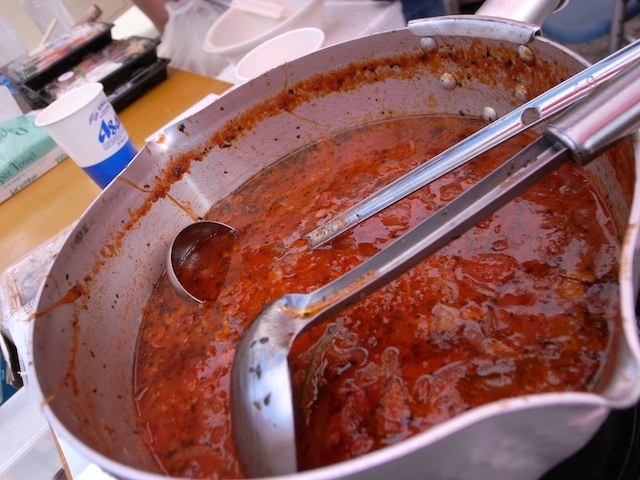The image depicts a white bowl, characterized by a curved front designed for pouring. Inside the bowl is a chunky red substance that appears to be either a tomato-based soup or sauce. The bowl is roughly half full, with a visible red ring indicating where the sauce or soup level used to be. Two silver ladles are placed inside the bowl; the larger ladle is face down, while the smaller one is facing up, with its handle extending out of the frame to the right. The scene is slightly tilted to the right.

In the background, on the left side of the image, there is a blue and white cup featuring the letters "ASA," positioned on a beige wooden table. Behind the cup are several black containers, presumably holding food, and some white buckets. Other indistinct items can also be seen, though they are somewhat blurred. The entire setup appears to be on a round countertop.